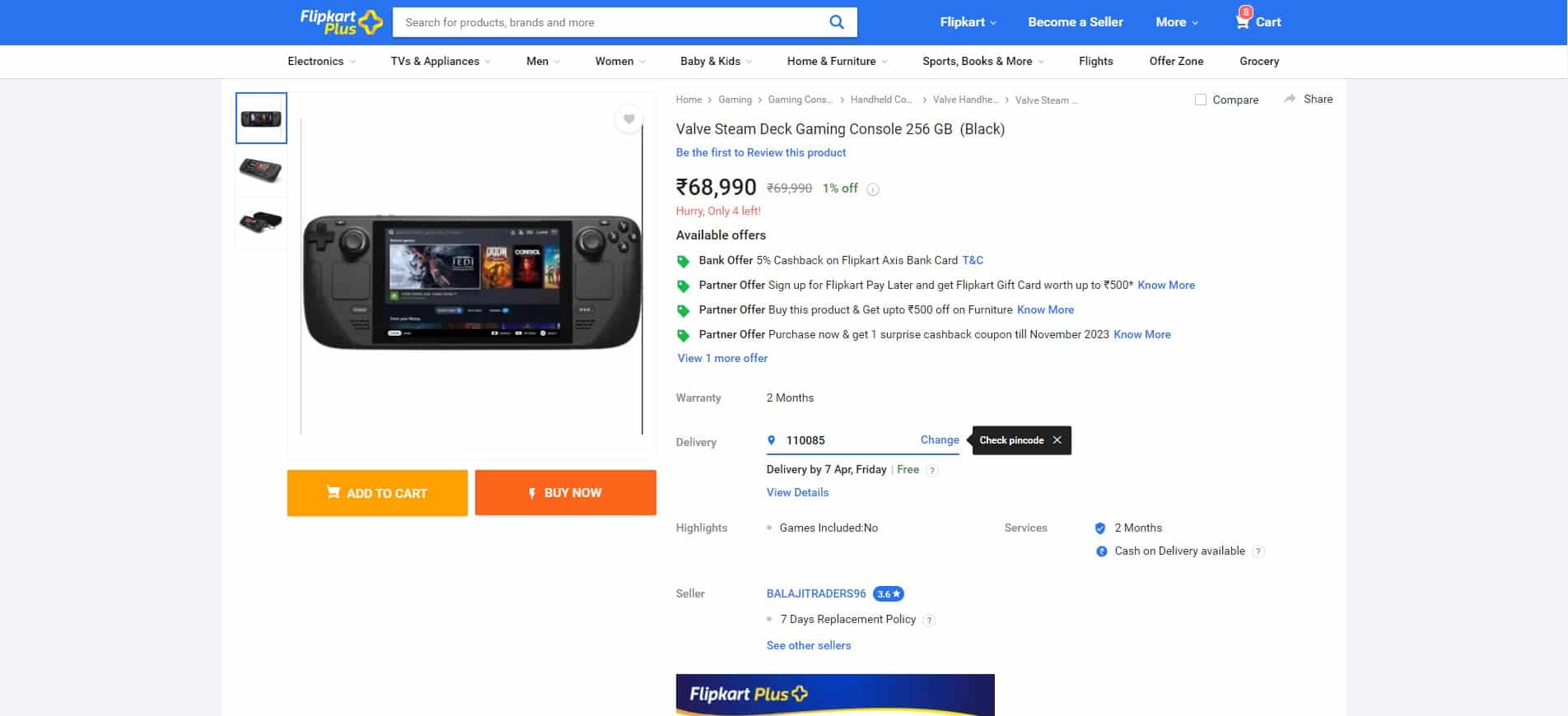This is a detailed monitor screen capture of a user's session on the Flipkart Plus website. The horizontally-positioned blue banner at the top prominently features the "Flipkart Plus" logo, with "Flipkart" in white and "Plus" in yellow, accompanied by a yellow plus sign to the right. Centrally located is the search bar, displaying a placeholder text: "Search for products, brands, and more." 

On the right side of the banner, there is a navigational menu comprising sections for "Flipkart," "Become a Seller," "More," and a "Cart" icon. The cart icon is highlighted with a red oval displaying a white numeral '8', indicating eight items in the cart.

The main focus of the screen is the listing for the Valve Steam Deck gaming console, featuring a 256 GB storage in black. Positioned against a white background, this gaming console listing is detailed on the right-hand side. The text “Be the first to review this product” is displayed in blue. The price is noted in a foreign currency as ₹68,990, with a small note indicating a 1% discount. In bold red text, it alerts users to "Hurry, only 4 left!"

Below the price, a series of available offers are listed, each marked with a green price tag icon:
1. Bank Offer: 5% cashback on Flipkart Axis Bank Card.
2. Partner Offer: Sign up for Flipkart Pay Later.
3. Partner Offer: Buy this product and get up to ₹500 off on furniture.
4. Partner Offer: Purchase now and get one surprise cashback coupon until November 2023.

Additional product specifics include a two-month warranty and an option to choose the delivery date. The note "Games included: No" highlights that no games come with the purchase. The seller, "Balazsit Traders 96," has a rating of 3.6 stars, accentuated by a blue oval. There is also a mention of a 7-day replacement policy and a prompt to "See other sellers."

To the left, multiple images of the Steam Deck are displayed, offering three different viewing options. Beneath the image window, there are two call-to-action buttons. The left button, light orange in color, displays an icon of a cart and the text "Add to Cart." The right button, darker orange with a lightning bolt icon, features the text "Buy Now" in white.

At the bottom of the screen, another blue banner with a yellow line displays "Flipkart Plus" branding.

Overall, this detailed screen capture provides an exhaustive view of the Valve Steam Deck product listing on the Flipkart Plus website, including product specifics, pricing, offers, seller information, and purchase options.